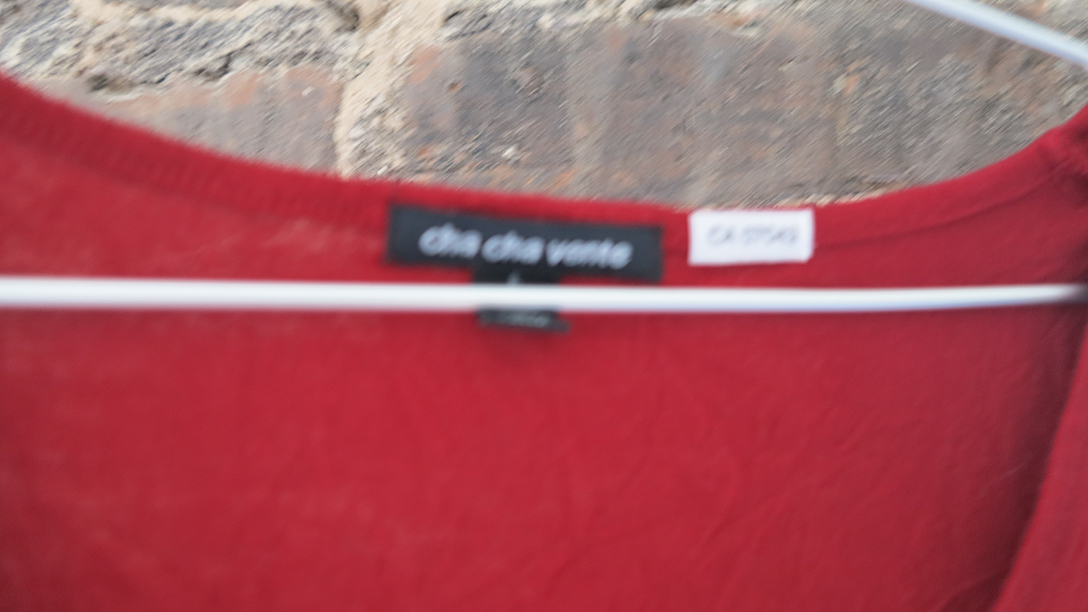This image is a close-up, somewhat blurry photograph featuring a red, long-sleeved dress shirt hanging on a white wire hanger. The shirt, prominently displaying a black rectangular designer tag with the brand name "Chachavente" embroidered in white thread, also features a smaller white tag beside it, which contains illegible green writing. Additionally, a smaller black tag with washing instructions and possibly the size, denoted by a white "S", hangs from the designer tag. The background reveals a deteriorating brick wall with visible chips and cracks in various shades of red, gray, orange-pink, and light beige.